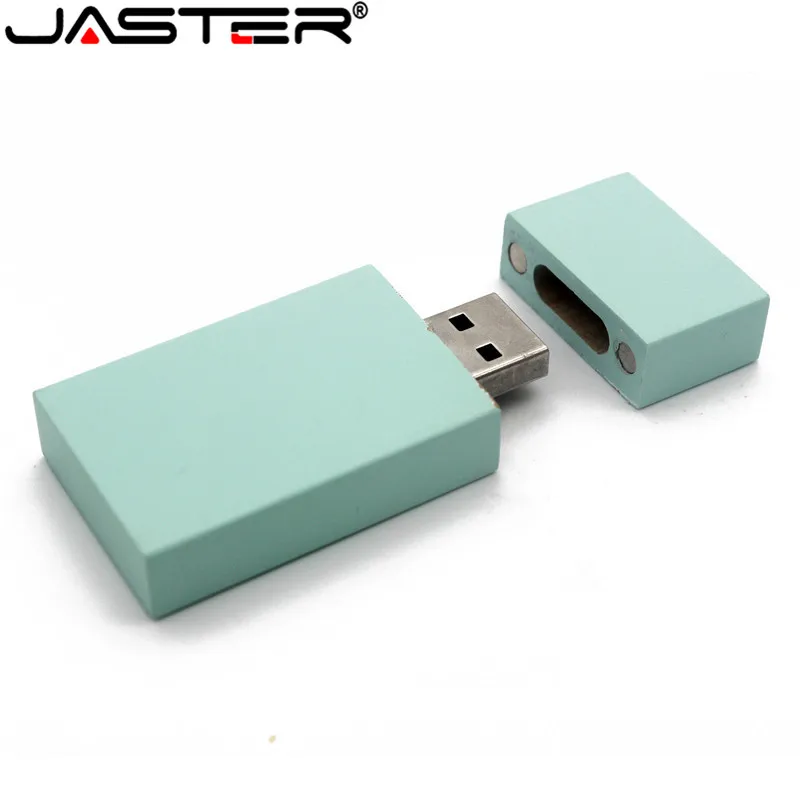This detailed product photo features a rectangular USB flash drive in a light seafoam green, or minty matte turquoise color, placed against a white background that emphasizes its simple and sleek design. The USB drive, angled at roughly a 45-degree angle with the right side elevated, displays a distinctive branding element at the top left corner where the brand name 'JASTER' is printed in black capital letters, with red accents inside the 'A' and 'E'. The metal USB connector, silver in color, is visible as the matching cap, slightly separated, shows two metal circles—likely magnets—underneath, hinting at a secure magnetic closure mechanism. Soft shadowing along the edges of the drive adds depth, making the product stand out visually.